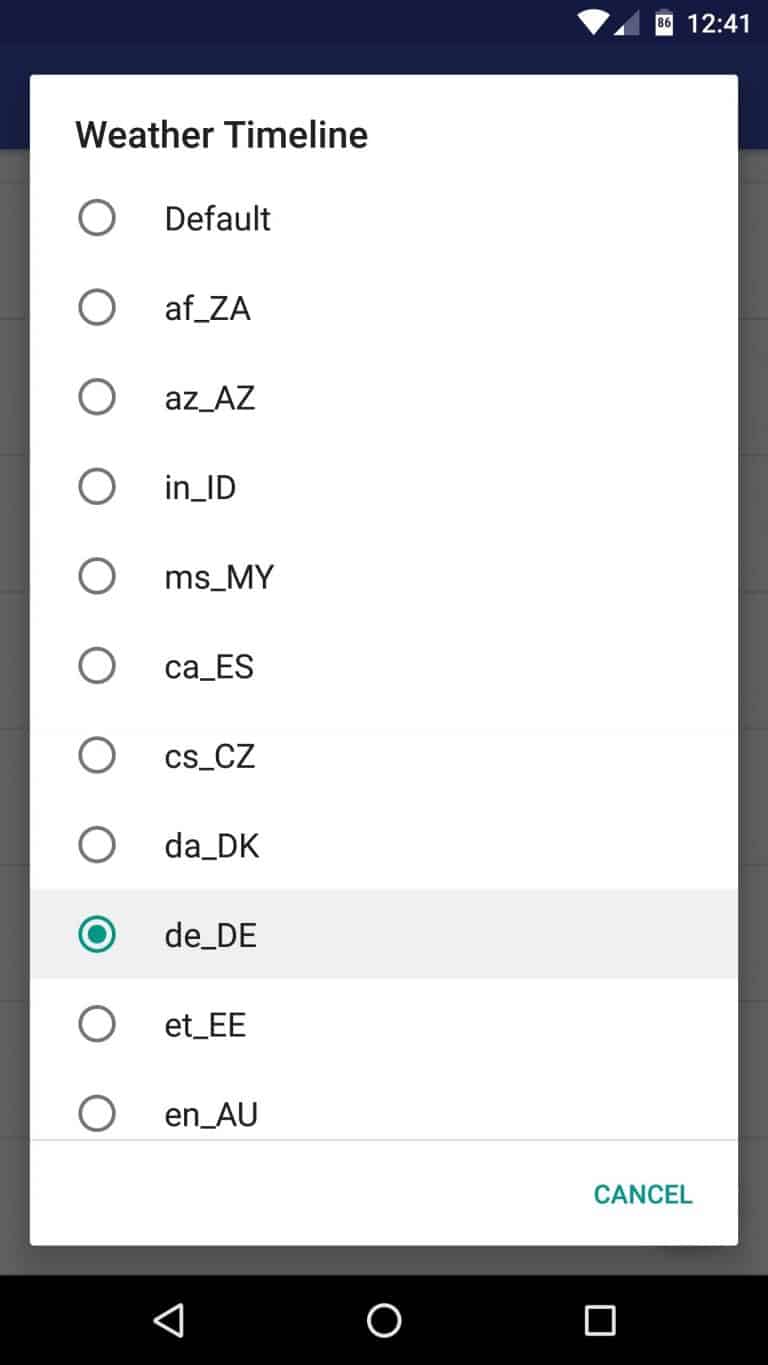In the image, there is a vertical box outlined in dark blue that transitions to dark gray. In the upper left corner, the time is displayed as 12:41, and the battery icon, in white, shows less than half charge. Inside the white square at the top, the text reads "Weather Timeline." 

Adjacent to this text is a circle with the label "Default." Below that, there is another line with a circle labeled "AF-ZA." The subsequent lines feature various two-letter codes paired with each other: "AZ-AZ" (with the second "AZ" capitalized), "IN-ID," "MS-MY," followed by "CA-ES," "CS-CZ," "DA-DK," and a highlighted gray circle with a green border denoted as "DE-DE." 

Following this, an empty circle is labeled "ET-ET." In the final row, a circle labeled "EN-AU" (both AU capitalized) is also present. 

In the bottom right corner, the word "Cancel" is displayed in green text. At the very bottom of the box, a long black bar features a central circle and a square to the right.